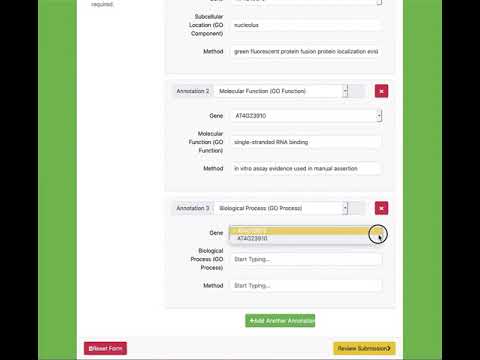This is a detailed screenshot from an unidentified application, lacking any clear indication of the app's name or the platform it operates on. The image is framed by a black bar along the top, followed by a green bar beneath it. The main content area features a white screen in the center. Within this white section, there are three distinct dialogue boxes displaying text that is too small to be comfortably read. Each dialogue box comprises at least three text entry fields, with one box labeled "Method," another possibly labeled "Biological Process," and a third potentially labeled "Gene." The purpose or functionality of the app remains unclear, leaving its exact use open to interpretation.